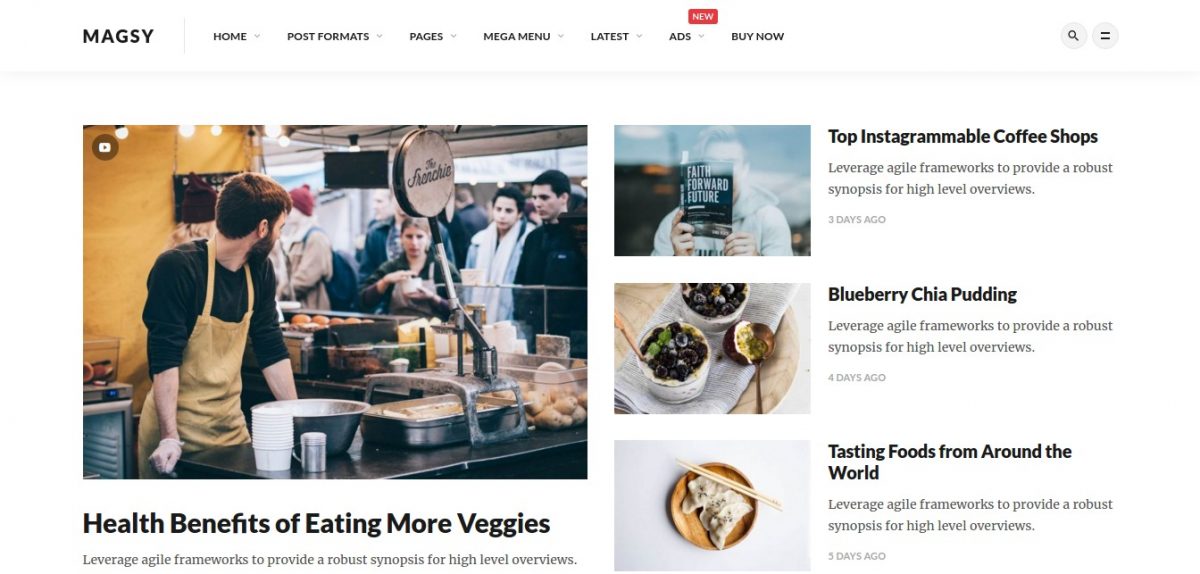Screenshot of a website with a white background. The website's top navigation bar includes the tabs: "Majesty," "Home," "Post Formats," "Pages," "Media," "Mega Menu," and "Latest Ads." Below the navigation bar, there are two circular icons; one features a magnifying glass indicating a search function, and the other has two overlapping rectangles likely representing a menu or a grid view option.

The main content of the screenshot showcases an image of a man in a bustling kitchen, surrounded by customers, emphasizing a lively and crowded atmosphere. The image is accompanied by the headline: "Health Benefits of Eating More Veggies."

To the right, a sidebar displays three smaller images with respective headings and timestamps. 
1. The first image promotes "Top Instagrammable Coffee Shops" with the repeated text "Leverage agile frameworks to provide a robust synopsis for high-level overviews." This post is marked as having been published "Three days ago."
  
2. The second image highlights "Blueberry Chai Pudding" with the same repeated subtext and is noted as "Four days ago."

3. The third image showcases "Tasting Foods from Around the World," again with the recurring subtext, marked "Five days ago."

Each small image underscores the central theme of leveraging agile frameworks to offer concise summaries for broad overviews.